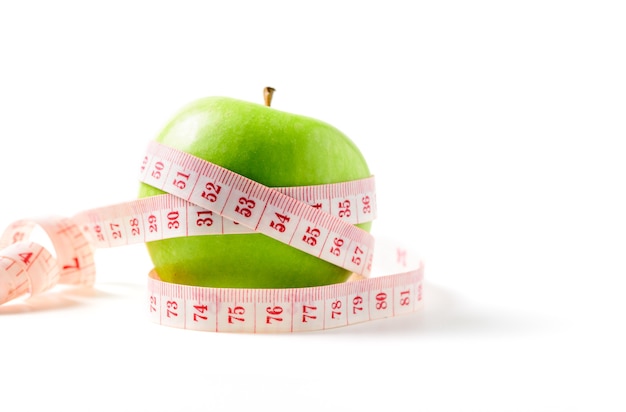In this well-lit photograph, a vibrant Granny Smith green apple takes center stage. The apple, sporting a small brown stem at the top, is meticulously wrapped with a flexible white sewing measuring tape. The tape, approximately half an inch wide, is marked by distinctive red numbers in a cursive or gothic style with elaborate curls, notably on the number "5". The measuring tape wraps around the apple three times: once at the base and twice criss-crossing in the middle, forming an X-shape that prominently showcases the numbers 73, 281, 50, 57, 36, 29, 4, and 7. The entire scene is set against a stark white background and surface, creating a minimally designed yet striking composition that highlights the green apple and the colorful, detailed tape.